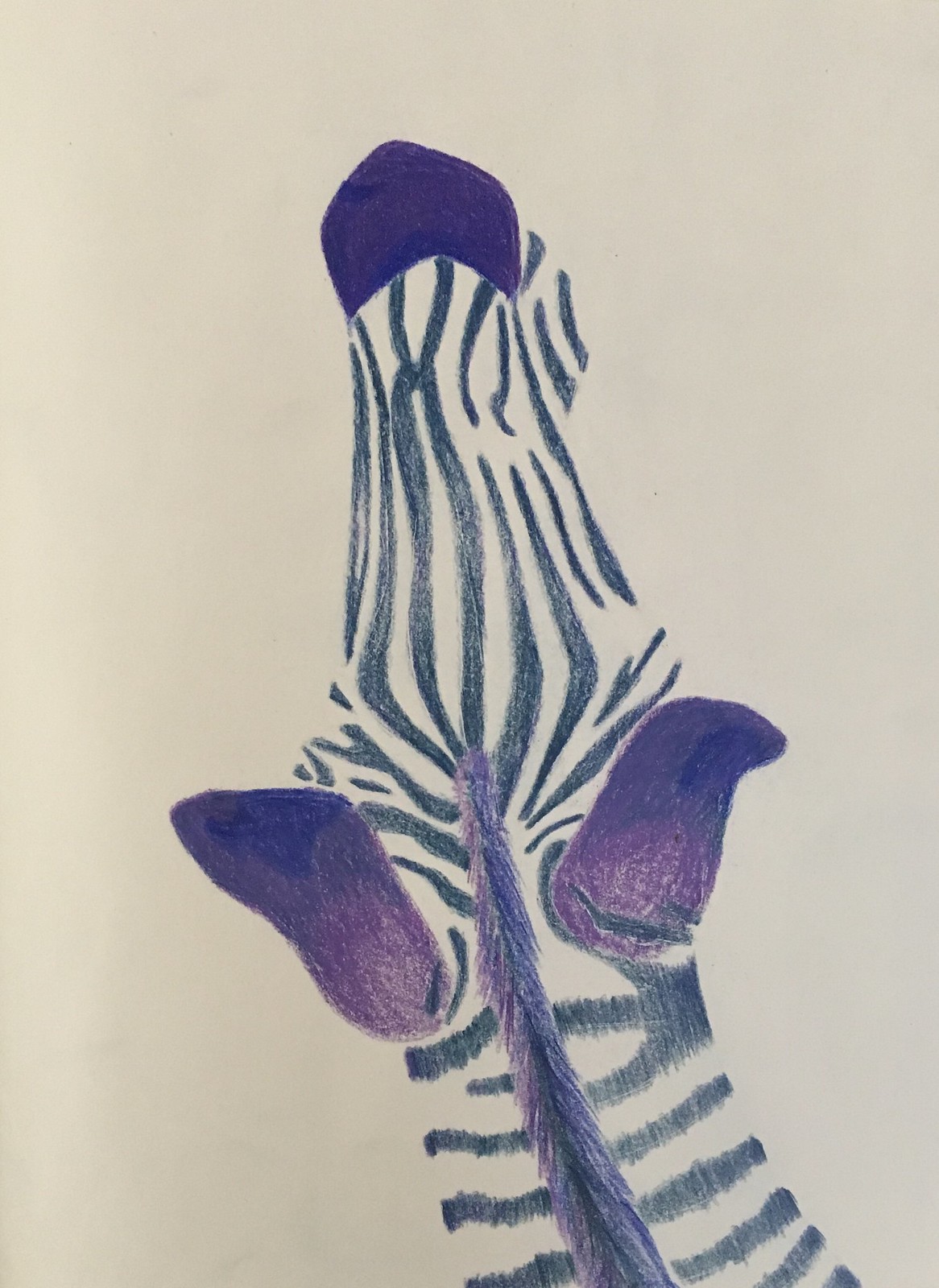This detailed photograph of a painting showcases a unique rendition of a zebra's head and neck, predominantly capturing the top-down perspective. Executed on cream-colored drawing paper, the artwork replaces the zebra's traditional black and white palette with a striking combination of purples and blues. The nose displays a bluish-purple hue with accents of violet, mirrored by the ears which contain more violet and splotches of dark blue. The mane is painted in vibrant purple with streaks of dark blue and violet, replacing the usual black hair. The customary black stripes are transformed into a dark blue, arranged in an irregular horizontal and vertical pattern across the visible portions of the zebra's head and upper neck. The stripes, described as having a charcoal color with lighter and darker shading to indicate depth, extend down below the nose. The careful detailing in the stripes and fur patterns, as well as the unconventional color choices, adds depth and artistic intrigue to the painting. While the eyes are not visible, the distinctive top-down perspective makes it unmistakably recognizable as a zebra.